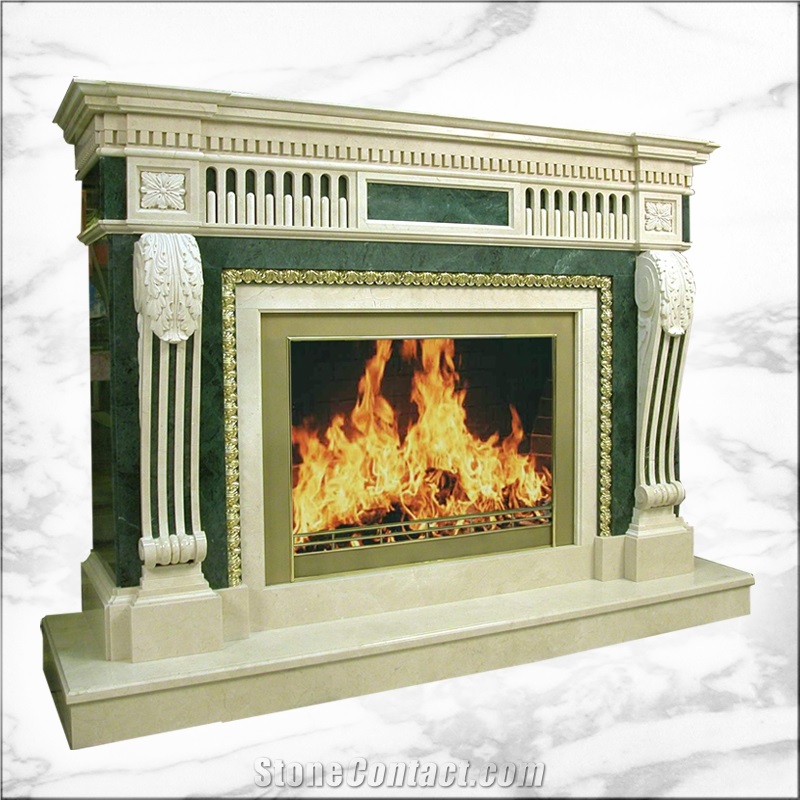The image appears to be a detailed, rectangular advertisement for a luxurious fireplace, framed by a thin black line. The background mimics a gray and white marble texture, providing an elegant backdrop. Dominating the center is a grand fireplace angled slightly to the right. This magnificent piece features a light tan concrete base supporting a dark green, marble-encased firebox. The fire appears to be lit, though it might be an edited effect. Above the firebox is a scrolling, ornate white design, with additional white detailing reminiscent of a Roman cathedral. This includes columns with spaces between them and a prominent horizontal green rectangle flanked by gray concrete squares. Throughout the design, there's a harmonious combination of white, gray, and various shades of brown, enhancing its Roman architectural charm. The image is branded with the site stonecontact.com subtly at the bottom.